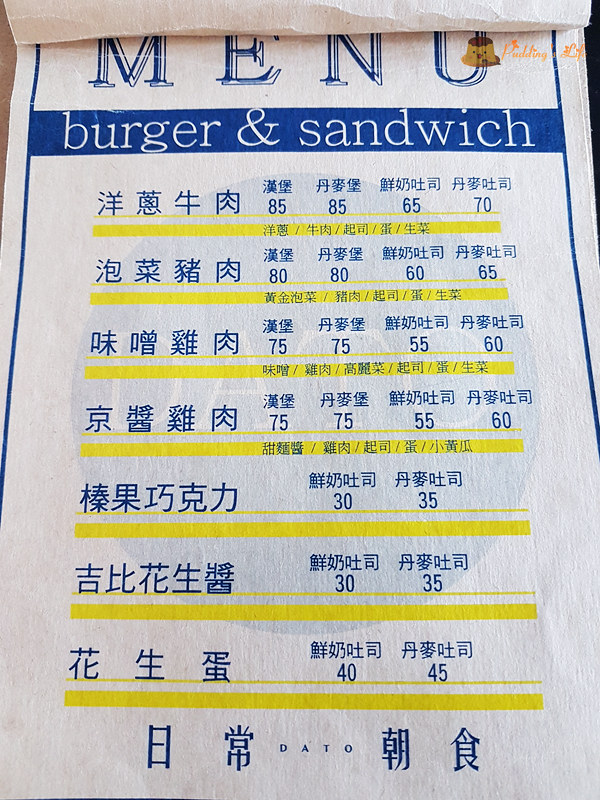This image depicts a poster likely hung on a wall, featuring a menu in both English and Chinese text. The English headings list types of food such as "burger" and "sandwich," while the accompanying Chinese descriptions provide more detailed information about the menu items. 

The poster is divided into sections, with the first four items each described by four Chinese characters, the last of which signifies "meat." Beneath each primary menu item, there are four additional descriptive lines, each accompanied by a different price, suggesting variations in size or style for each item.

Notably, all further descriptive lines are uniform across the items, indicating a consistent categorization perhaps related to portion sizes, preparation methods, or ingredient options. Towards the bottom of the poster, a line of Chinese text features the term "DATO" written in Western characters, though its meaning remains unclear.

The poster's overall layout is organized and methodical, aiding in easy comparison of options despite the language barrier for non-Chinese speakers.